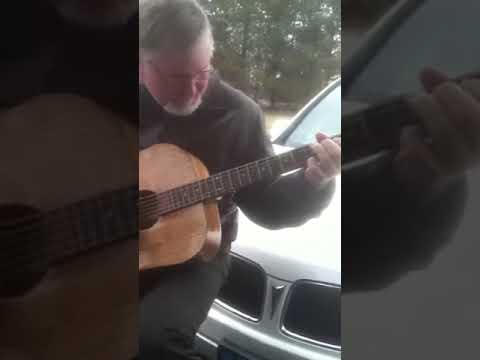In this detailed outdoor scene, an older man with glasses, characterized by his graying dark hair and a grayish-white goatee, is captured playing a well-worn, two-toned brown guitar. He is positioned on the left side of the vertical image and is leaning against the hood of a silver car, resembling a compact SUV with indistinguishable front grille logo and metallic silver accents. Dressed in a potentially dark gray or light black long-sleeve shirt and dark pants, he strums the guitar with his fingers on the fretboard while his left leg is arched up to support the instrument. The man’s face has a reddish hue, suggesting he is Caucasian. In the background, the setting reveals a heavily wooded area with green leaves peeking through, indicating a daytime, outdoor setting. The image is framed with black bars on each vertical end, creating a partial translucent view of the surroundings. The overall color palette includes black, tan, brown, silver, gray, green, and light green, giving depth to the natural and serene environment.